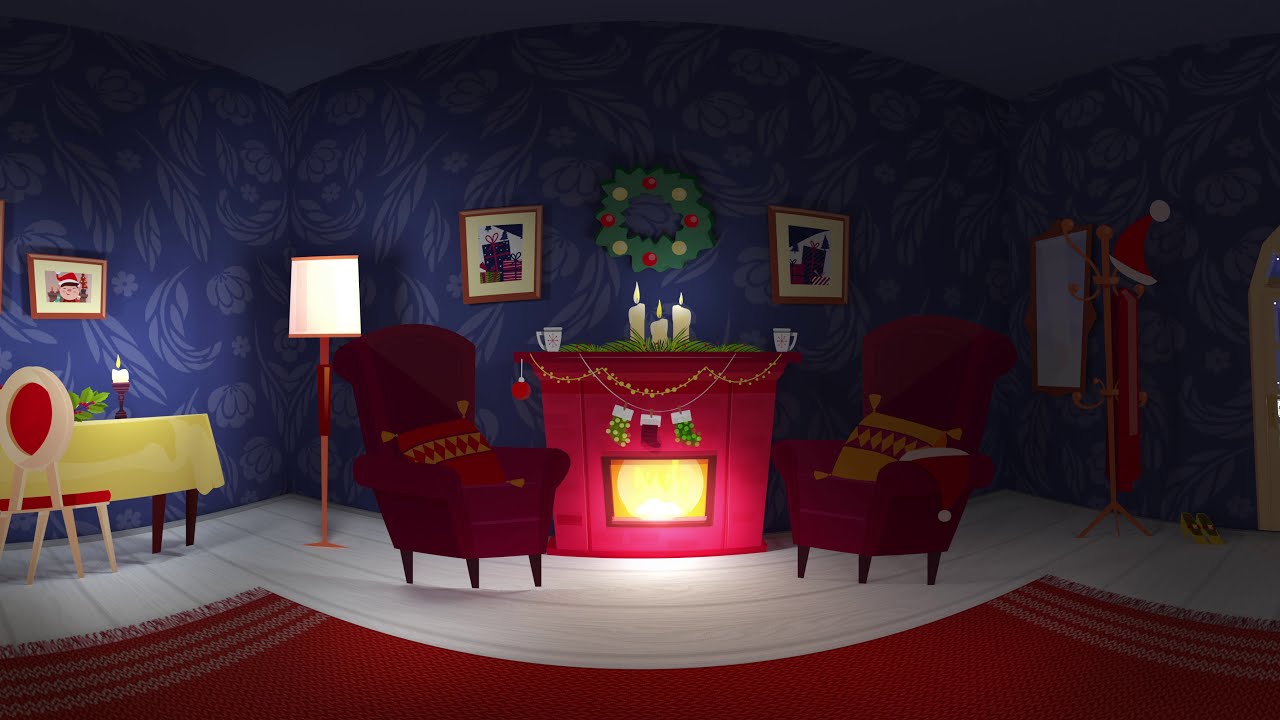The image depicts a charming, computer-generated, panoramic view of an animated, Christmas-themed living room. The slightly distorted panoramic shot reveals a cozy environment reminiscent of a scene from virtual reality. The walls are adorned with dark blue floral wallpaper featuring lighter blue leaf patterns. Central to the room is a red fireplace, brightly lit with a roaring fire, adorned with glowing candles on the mantelpiece, and hung with festive stockings and garlands. Above the mantle hangs a green Christmas wreath, flanked by two portrait photos, one of which depicts an elf or Santa. Two overstuffed chairs, each accompanied by checkered pillows in red and orange, are positioned on either side of the fireplace. The chair on the right hosts a Santa hat draped over its arm. Behind this chair stands a coat rack adorned with another Santa hat, next to a doorway and a mirror. The left side features a small table and a floor lamp behind the chair. A lush, red rug covers the floor, enhancing the room’s festive atmosphere. The entire scene is softly lit by the warm glow emanating from the fireplace, creating a cozy and inviting holiday ambiance.